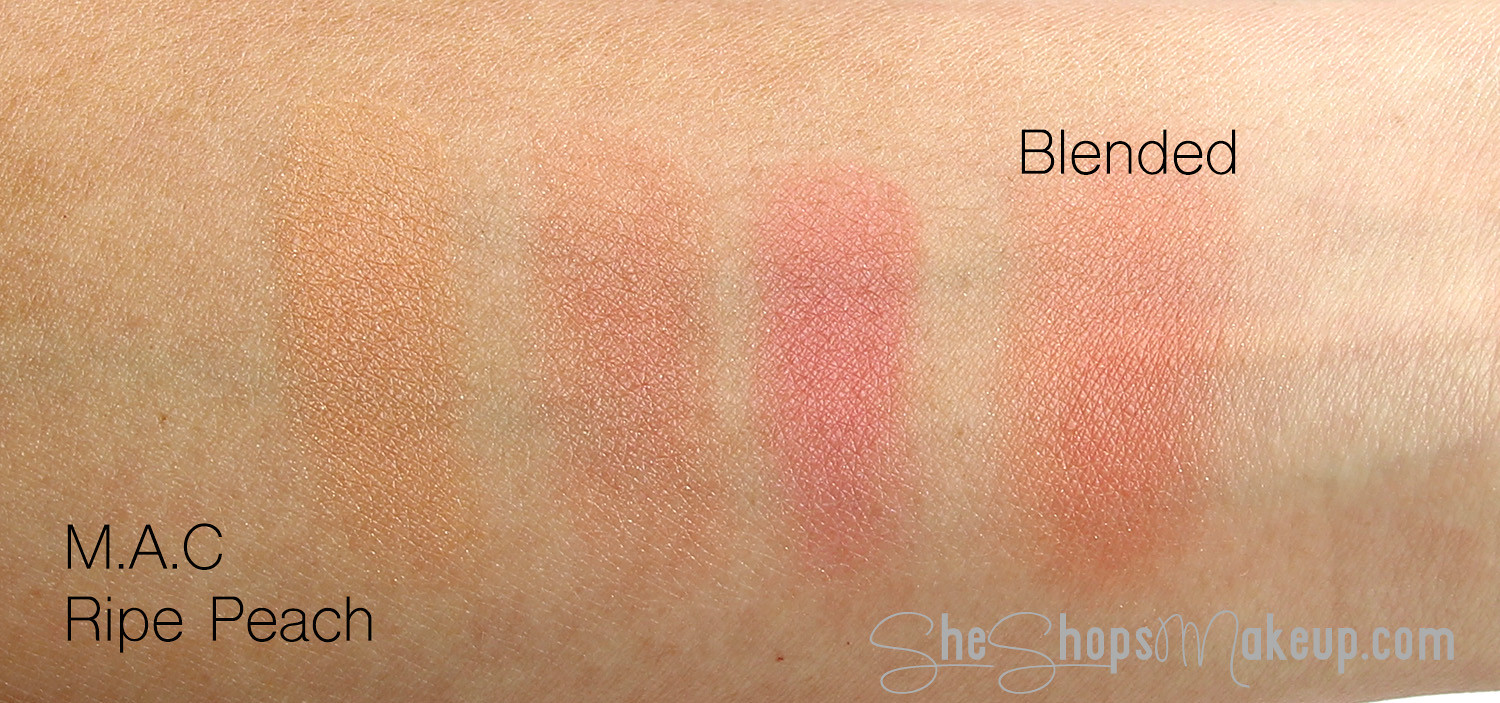This close-up advertisement photo showcases a Caucasian person's inner forearm with detailed, visible skin lines. Four distinct swabs of makeup are applied: a cream color on the left, advancing to dark red, then a pastel, vibrant reddish-pink, and finally an orange hue on the right. The second swab is labeled "MAC ripe peach" in black text at the bottom left, and the fourth swab is noted as "blended" in black text above it. In the bottom right corner, the website www.SheShopsMakeup.com is displayed in blue script. The image meticulously highlights the different makeup colors and their application on the skin, emphasizing the texture and color contrast.